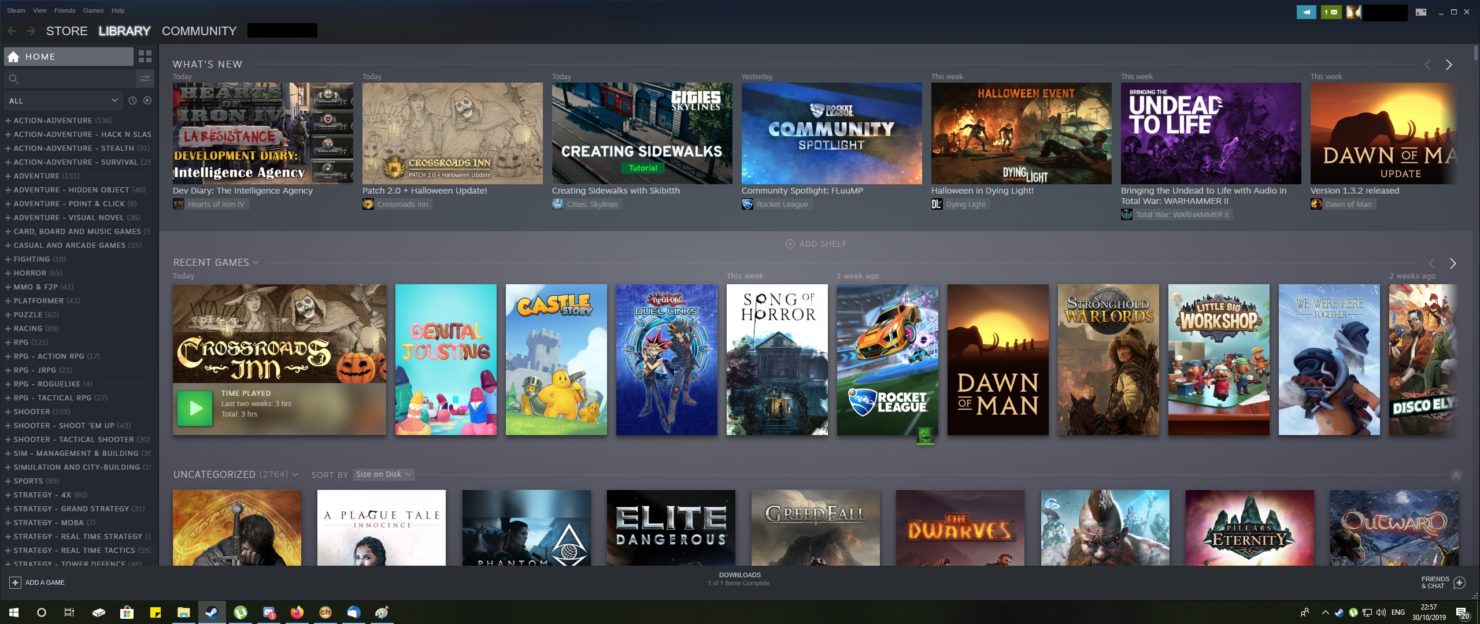This screenshot appears to be from a digital game library interface. In the upper left corner, there are headers labeled "Store," "Library," and "Community." To the left, a table lists various games, organized alphabetically, with a search bar featuring a magnifying glass icon at the top. The background is predominantly black, giving a sleek and modern look to the interface.

The main section of the webpage showcases games, arranged in three visible rows, each displaying several game titles with corresponding cover art. Although the font size is small, making it challenging to read the titles, the top row includes: "Intelligent Agencies," "Grossling Inn," "Creating Sideworks," "Community Spotlight," "Halloween Event," "Undead to Life," and "Dawn of Man." 

The middle row features: "Crossroads Inn," "Existential," "Castle," "Songs of Horror," "Rocket League," "Man of Dawn," "Warlords," and "Little Workshop," as well as "Disco Elysium." 

The bottom row, partially obscured, lists: "Plague Tale," "Elite Dangerous," "Greedfall," "The Dwarves," and "Turning Outwards."

Each game is accompanied by its cover art, adding visual interest. At the bottom of the screen, a series of icons represent various functions and applications, with additional icons located in both bottom corners, contributing to the comprehensive navigational design of the interface.